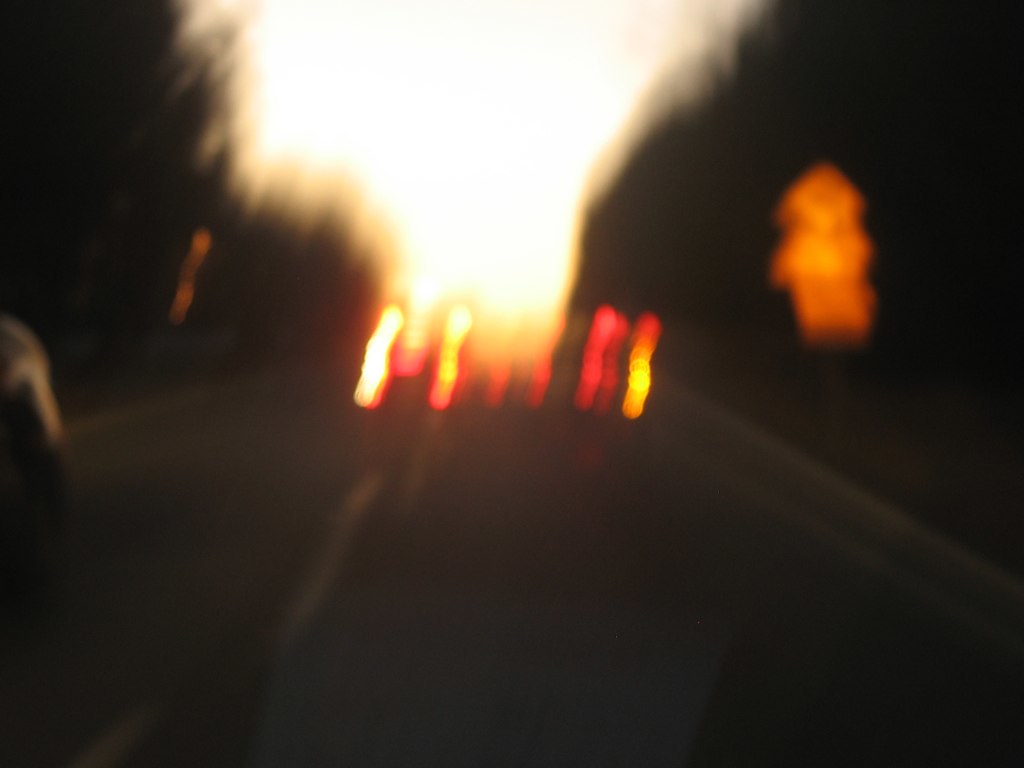The image portrays a very blurry scene, likely captured by someone behind the wheel. It shows a stretch of road ahead, framed by the car’s visor at the top. Two vehicles are visible in both lanes, viewed from behind with their red brake lights shining. Road signs appear on the right, though they are too blurred to discern any text. The sky is clear, but the low angle of the sun, either setting or rising, casts long shadows over the trees and forest on both sides of the road, creating a dim and shadowy ambiance.